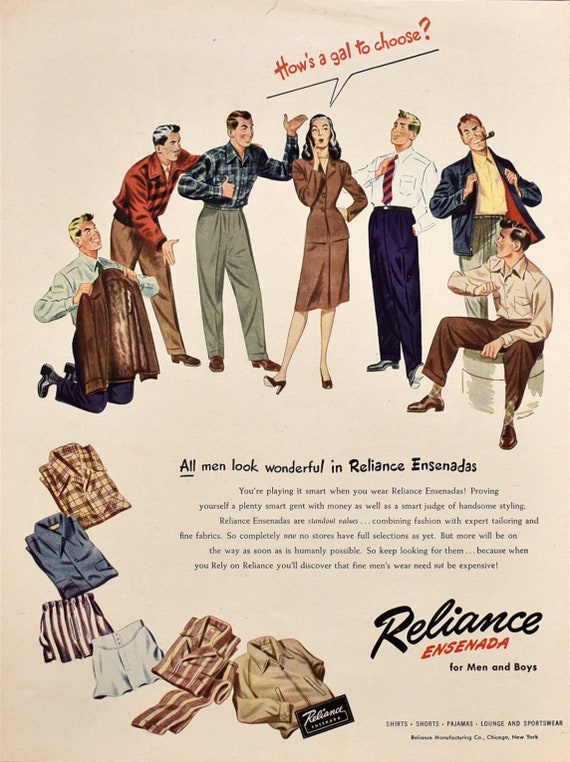The advertisement appears to be a vintage, 1950s or early 1960s styled illustration for a men’s clothing line called Reliance Ensenada, targeted at "men and boys." Central to the image is a woman in a brown skirt suit with black hair, depicted with one foot up in the air, and a hand on her chin. A speech bubble above her head reads, "How's a gal to choose?" She is flanked by six men, three on each side, all vying for her attention and showcasing different Reliance Ensenada outfits. 

The men’s attire varies: one man holds a jacket and kneels; another in a red shirt and khakis spreads his arms; a third in gray pants and a blue checkered shirt gives a thumbs up. On the other side, a man in dark blue pants and a white shirt holds a red and black striped tie, another showcases his yellow button-down shirt and khakis by holding his blue jacket open while smoking a pipe, and the last man sits on a box wearing brown pants, argyle socks, and a light brown shirt, lifting his arm to highlight his attire.

The ad's text emphasizes that "All men look wonderful in Reliance Ensenada," with additional smaller text extolling the quality, fashion, and affordability of the garments. The overall background is beige, adding to the vintage aesthetic. The bottom right corner reiterates the brand with, "Reliance Ensenada for men and boys."